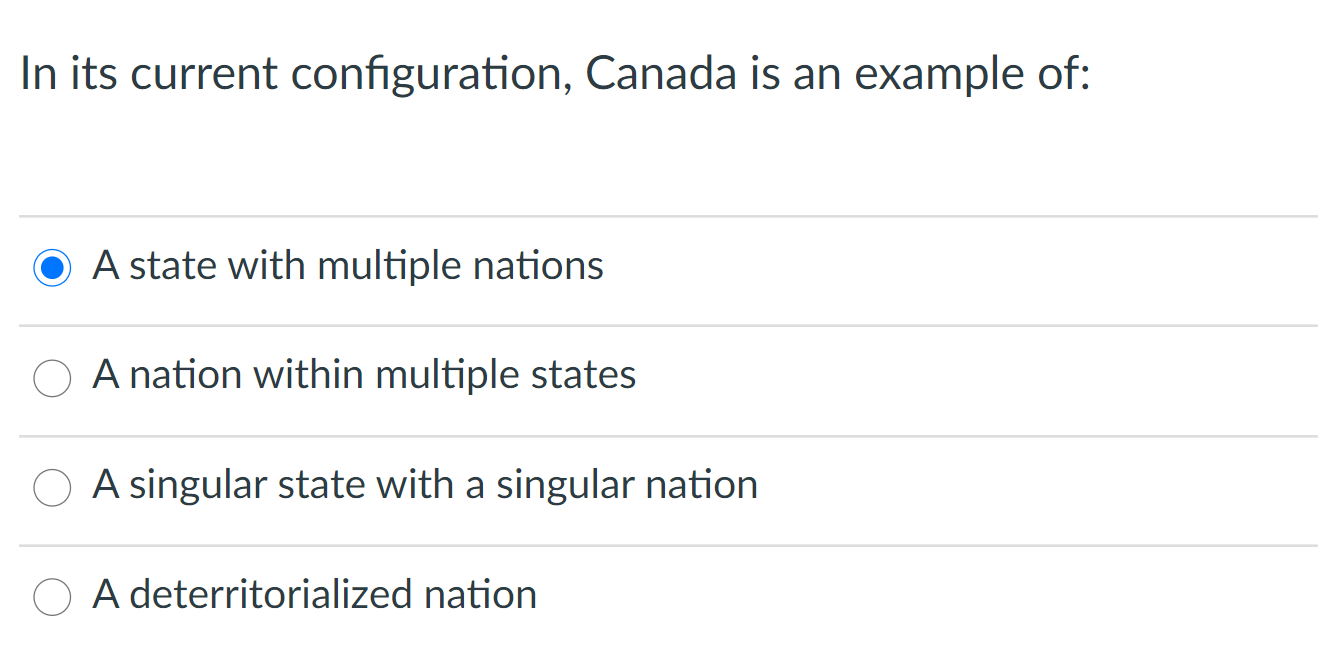The image features a multiple-choice question with a clean white background. The question, written in black text, reads: **"In its current configuration, Canada is an example of:"** Below the query are four options for the user to choose from:

1. **A state with multiple nations** (selected in blue)
2. **A nation within multiple states**
3. **A single state with a singular nation**
4. **A deterritorialized nation**

The first option is chosen, highlighted in blue to indicate selection. Each choice is separated by horizontal lines for clarity, creating a neat and organized format. The visual layout includes spaces to clearly distinguish the question from the answer choices, ensuring the text is easy to read and aesthetically balanced. The design resembles that of a standardized test, providing a straightforward and user-friendly interface for selecting answers.